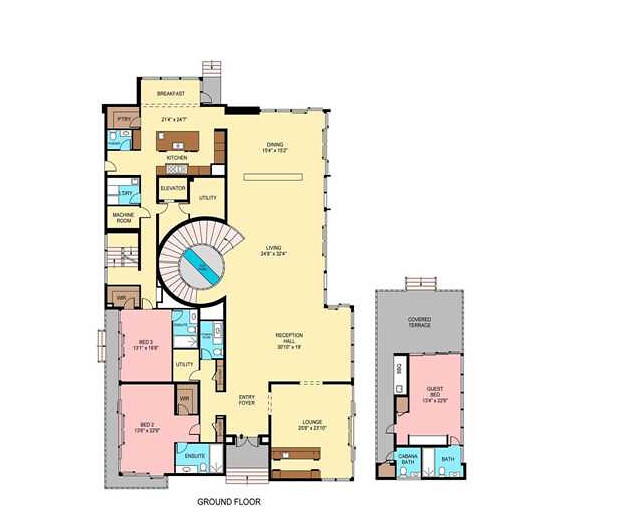This detailed diagram illustrates the floor plan of an expansive residential property, possibly an apartment or a house. The layout is presented in a large, square-shaped format with a prominent use of color to differentiate various sections. 

The largest section, highlighted in yellow, encompasses several communal areas, including a dining area, living area, reception hall, lounge (enclosed by walls), entry foyer, a prominently featured circular stairway, an elevator, kitchen, and machine room. These spaces are designed to facilitate daily living and social gatherings.

Adjacent to these communal spaces are designated bedroom areas marked in pink. This includes Bedroom 3, Bedroom 2, and a Guest Bedroom, each clearly labeled to indicate their function. Additionally, there are separate blue-colored sections indicating bathrooms, strategically placed to serve both the communal and private areas.

The diagram also includes an upstairs section, depicted in gray, featuring a rectangular Covered Terrace, which provides a versatile space possibly used for outdoor activities while being adjacent to the upper-level bedroom. 

Overall, this floor plan serves as a comprehensive visual representation ideal for prospective renters or buyers to understand the spatial distribution and functional areas within the property.